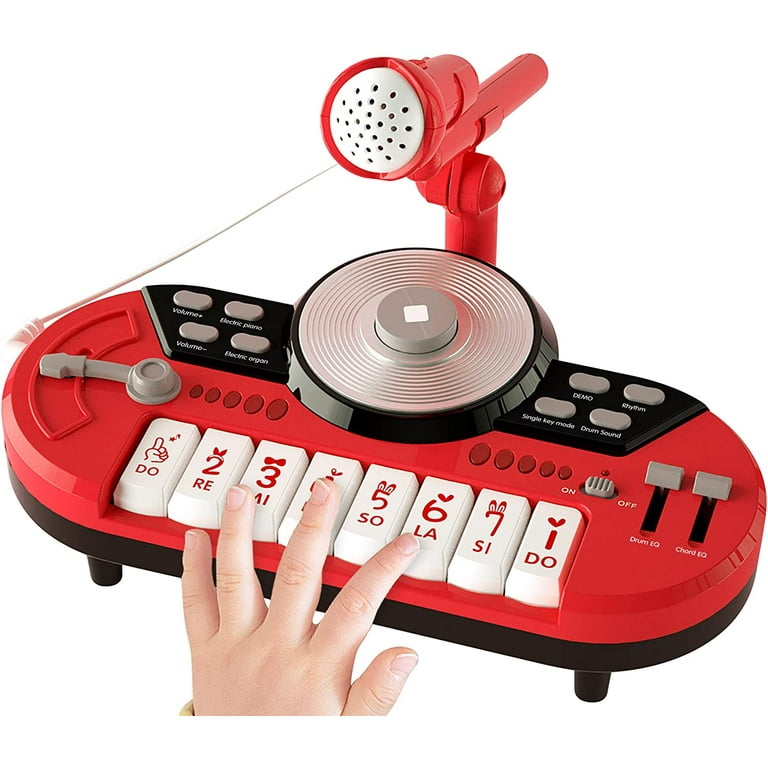This full-color, professionally staged photograph showcases an educational child's toy designed to teach music. The image features only the left hand of a very young, likely Caucasian child interacting with a piano-like device. The toy is predominantly red and silver, with white keys labeled "Do, Re, Mi, Fa, Sol, La, Ti, Do." These labels are accompanied by numbers 1 through 7 plus 1. The device also has various controls resembling those on a boombox, including volume levers, buttons, and switches, as well as a red microphone. The toy aims to mimic a DJ experience, allowing children to play and learn musical notes.